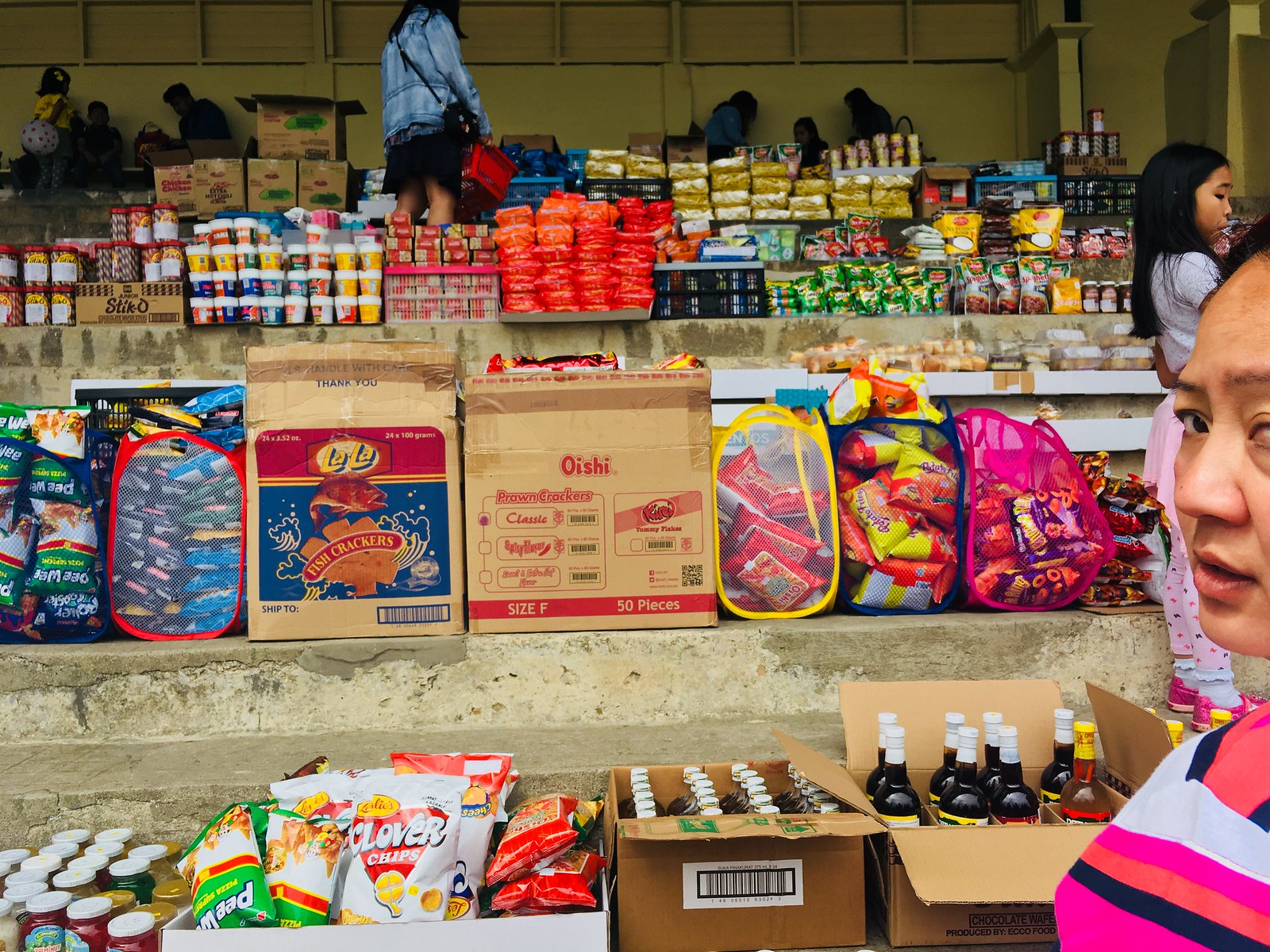The photograph depicts an outdoor Asian market, characterized by a bustling scene of people searching for goods among partially disorganized shelves and boxes. The shelves, which resemble worn cement steps, are stacked with various food items such as cardboard boxes of crackers, canned food, colorful packaged goods, jars, and tins, although some items are not easily identifiable. Among the shelves, there are open boxes that appear to contain some type of liquid. In the foreground, on the right side, a person is looking to the left, while a young female behind them gazes in the opposite direction. The atmosphere is lively, with around four individuals navigating through the market in search of food, amidst a diverse array of products displayed in vibrant packaging with text in different languages.